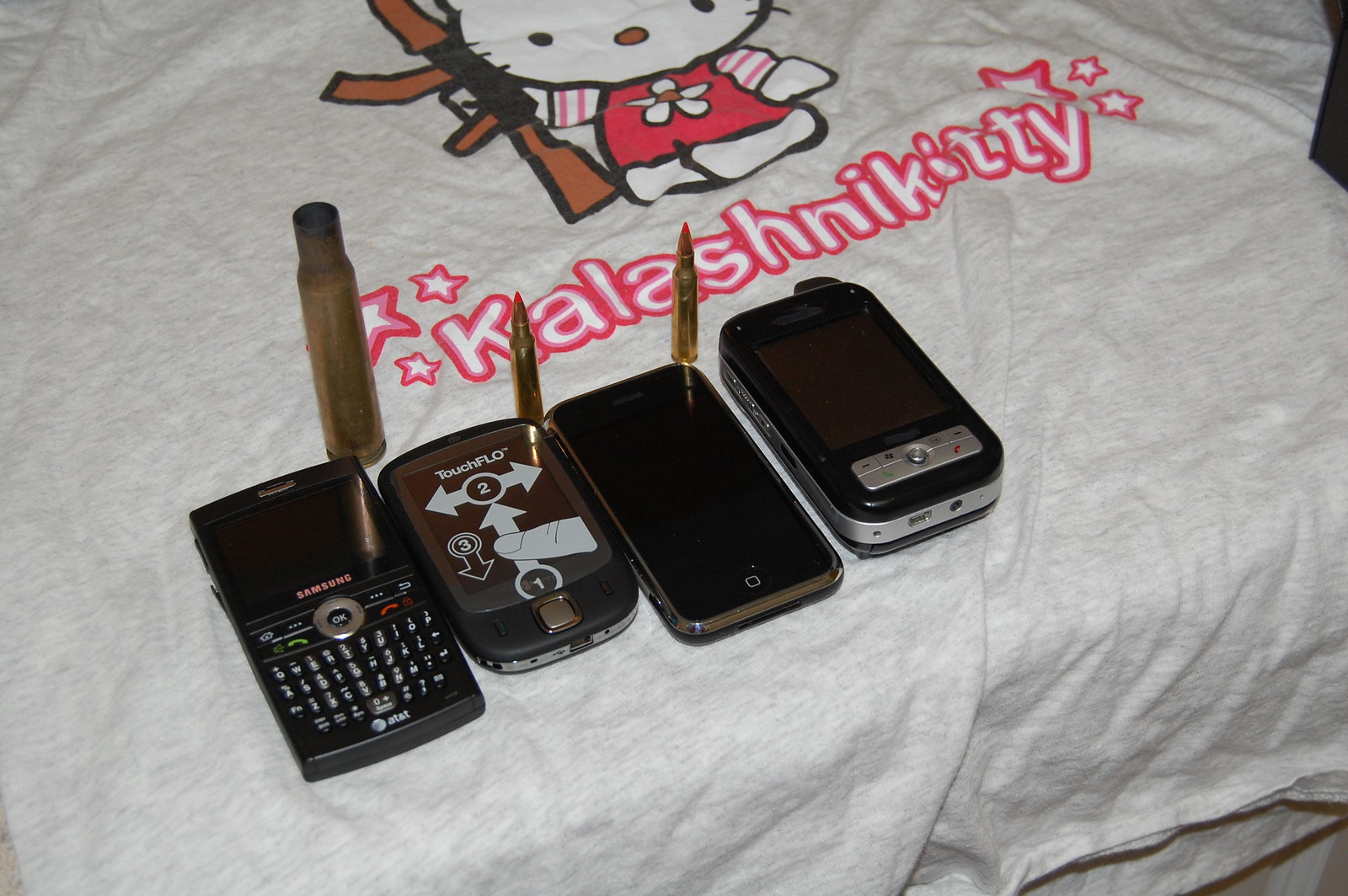The image depicts a white t-shirt draped over the edge of a table, showcasing a detailed and cutesy yet provocative illustration. The fabric features the iconic Sanrio character Hello Kitty, clad in a bright pink outfit adorned with flowers, but armed with a machine gun in her right hand. Below the character, the word "Kalashnikitty" is emblazoned in bold pink letters, flanked by small stars. Surrounding this text are a mix of electronic devices, including what appear to be early smartphones and remote controls. The first device displays the AT&T logo, and another indicates "Touch Flow" with directional arrows. Additional devices are less distinct. Positioned among these electronics are three large-caliber brass bullets: the first is an empty shell casing standing on end, while the other two are complete bullets, also standing upright. The juxtaposition of whimsical and menacing elements creates a striking and somewhat unsettling scene.